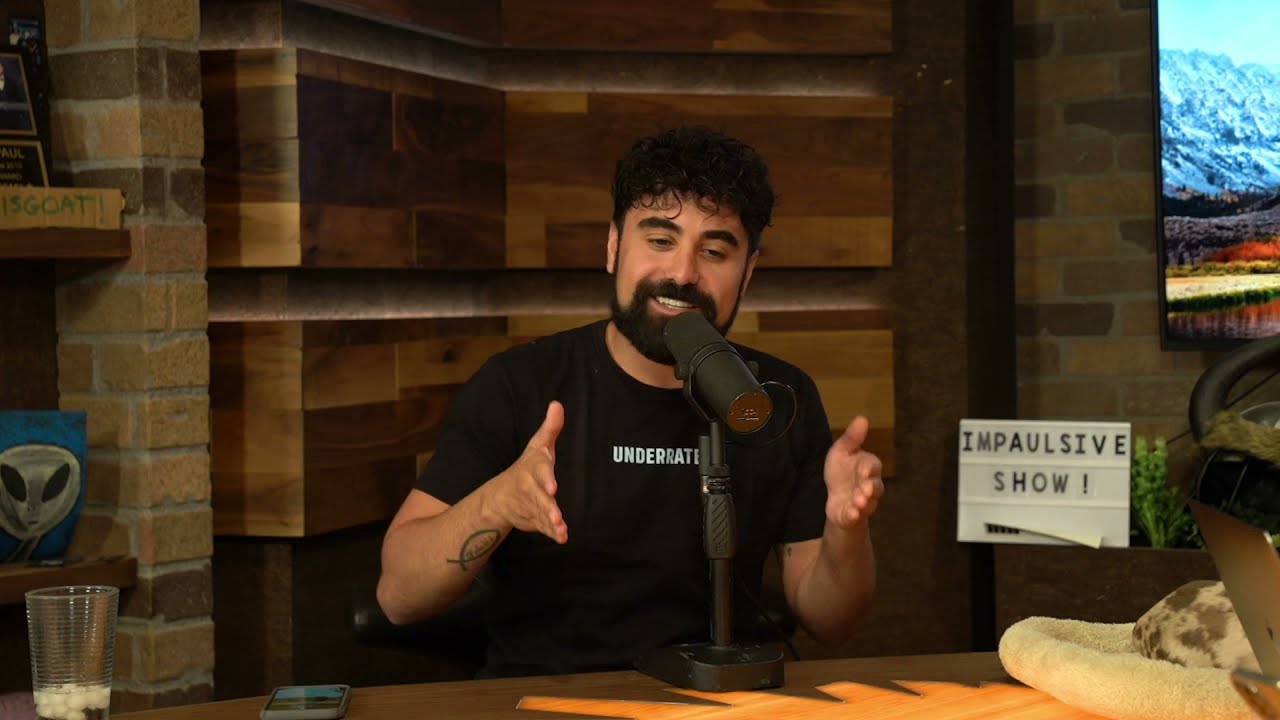In this photograph, a man in his early 30s sits at a wooden desk, engaging with a large, professional black microphone positioned in front of him. He has pale tan skin, black curly hair that's longer on top, a thick but short black beard, and pronounced bushy eyebrows. He is wearing a short-sleeved black t-shirt with the partially visible white, all-caps text "underrated." He sports a tattoo resembling a Christian fish symbol on his left forearm. His hands are extended forward as if gesturing, with fingers closed and thumbs up, as though holding an imaginary box. A nearly empty glass of water and a cell phone are placed on the desk. The background features a mix of wooden paneling and brick, creating a cozy, well-structured environment. There is a "IMPAULSIVE SHOW!" sign on a white board behind him, a corner shelf displays a small painting of an alien, and the top right corner shows part of a TV screen depicting a snow-covered forest landscape. The man is looking downward, slightly past the microphone, with a subtle smile on his face.